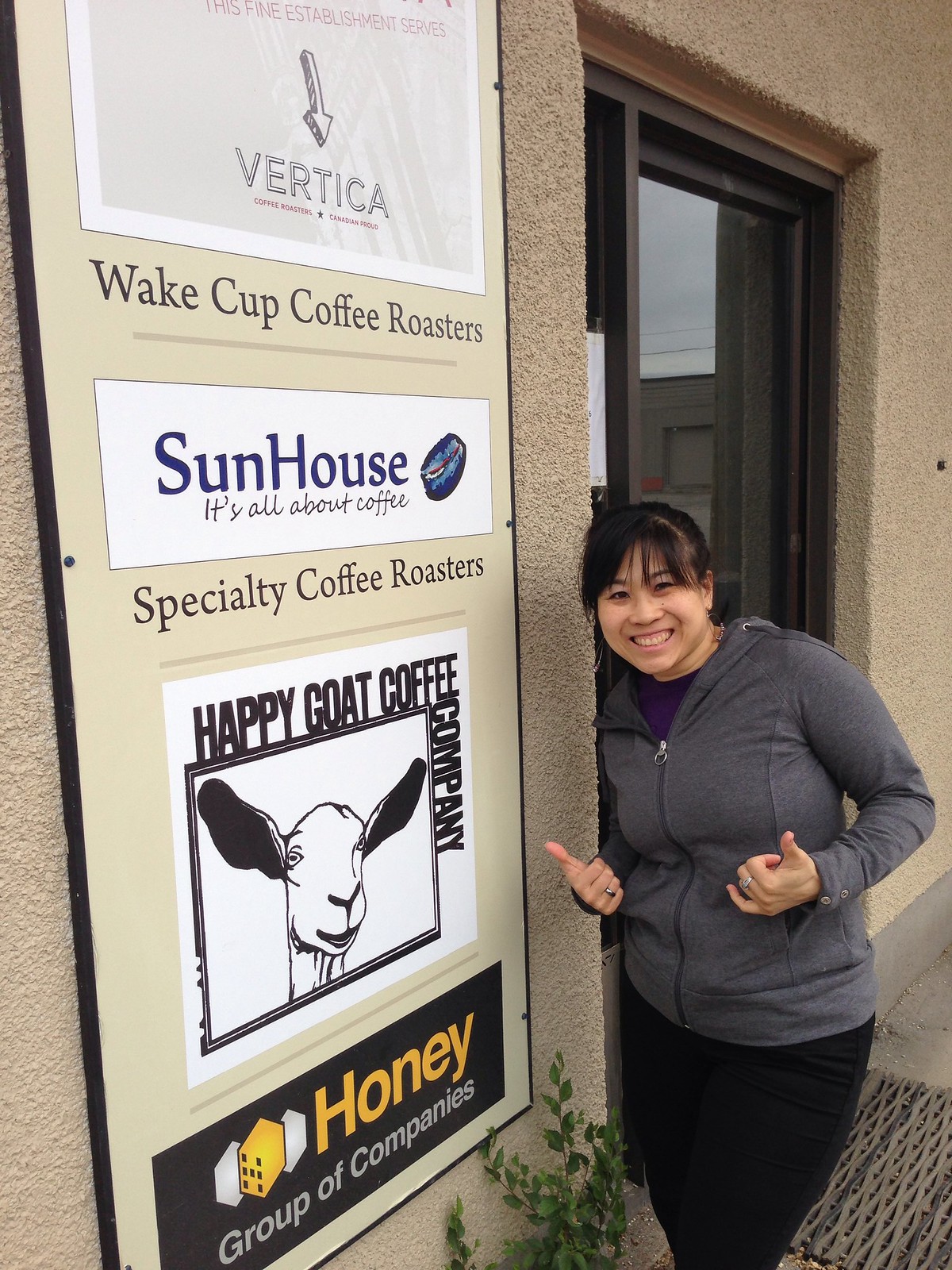The photograph captures a young Asian woman standing in front of a brown stucco building, leaning slightly against a wooden door framed with wood. She is dressed in a gray zippered jacket over a possible purple t-shirt, black pants, and is accessorized with a ring and earrings. Her short hair frames her smiling face, and she exudes confidence with both hands held up in a thumbs-up gesture. To her right, several signs are displayed. The top sign reads "Vertica", followed by "Wake Cup Coffee Roasters" printed in black on a beige background. Below this is a vertical white sign with blue writing that reads, "Sun House, It's All About Coffee," featuring an image of a coffee bean and the words "Specialty Coffee Roasters." Another sign features a black drawing of a goat encircled in a square with the text "Happy Goat Coffee Company," and at the bottom, "Honey Group of Companies." The scene suggests a setting associated with multiple coffee-related businesses.